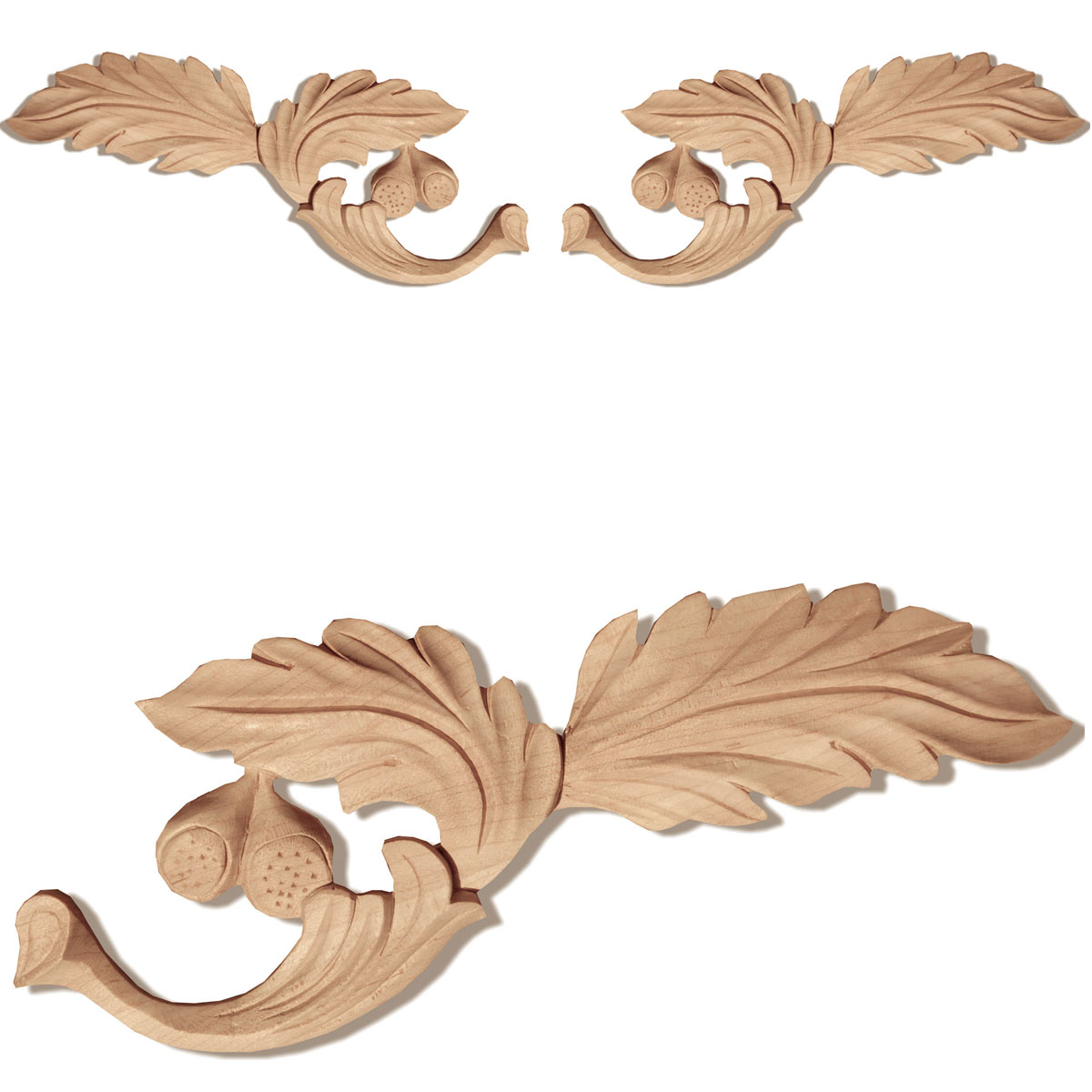The image features three intricately carved tan-colored wooden or ceramic decorative pieces set against a white background. Each piece is a depiction of a large leaf with detailed vein lines and a smooth, curved design. The two upper pieces are mirror images of each other, with one oriented to the left and the other to the right. They are connected by a U-shaped cascading leaf that adds a sense of flow to the composition. Hanging from the leaf on the right are two small, berry-like objects or nuts, potentially resembling acorns. Below these two is an enlarged, close-up view of the right-hand piece, showcasing the fine hand-carved details and the texture of the leaves. The overall artistry and angelic appearance of the leaves give an impression of them being freshly fallen, adding to the decorative charm.